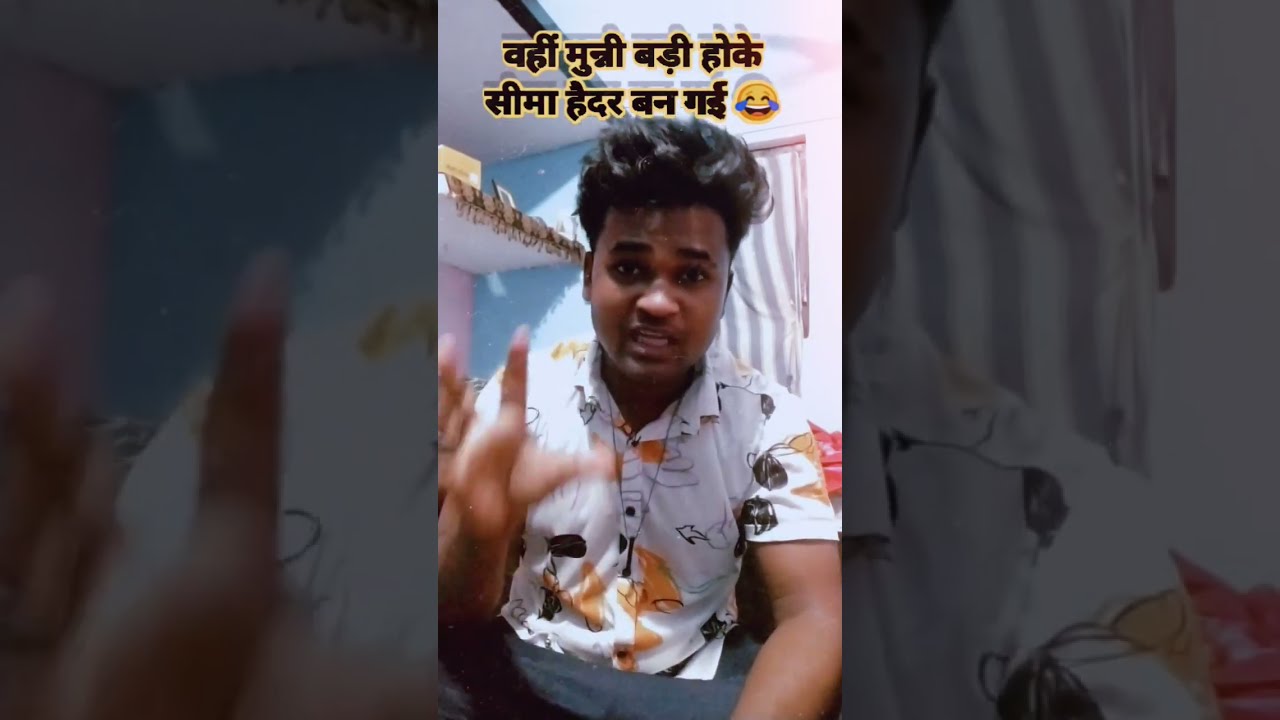The image is divided into three vertical sections. The middle section features a photograph of a young Indian boy with dark brown skin and poofy, black hair styled high off his head. He is sitting cross-legged inside a room with a low ceiling and is wearing a short-sleeved, collared white shirt adorned with orange and black designs. The boy appears to be speaking, his mouth open with his upper and lower teeth visible, and his right hand is raised as if to emphasize his words. In the background, there is a white shelf, light blue walls with some white patches, and a gray and white striped curtain covering a doorway. Above the boy's head is text in Hindi: وہیں منہ بڑی ہوکے سیما حیدر بن گئی, followed by a laughing emoji. The first and third sections of the image are blurred, darkened close-ups of parts of the photograph in the middle, serving as a border around the main image.